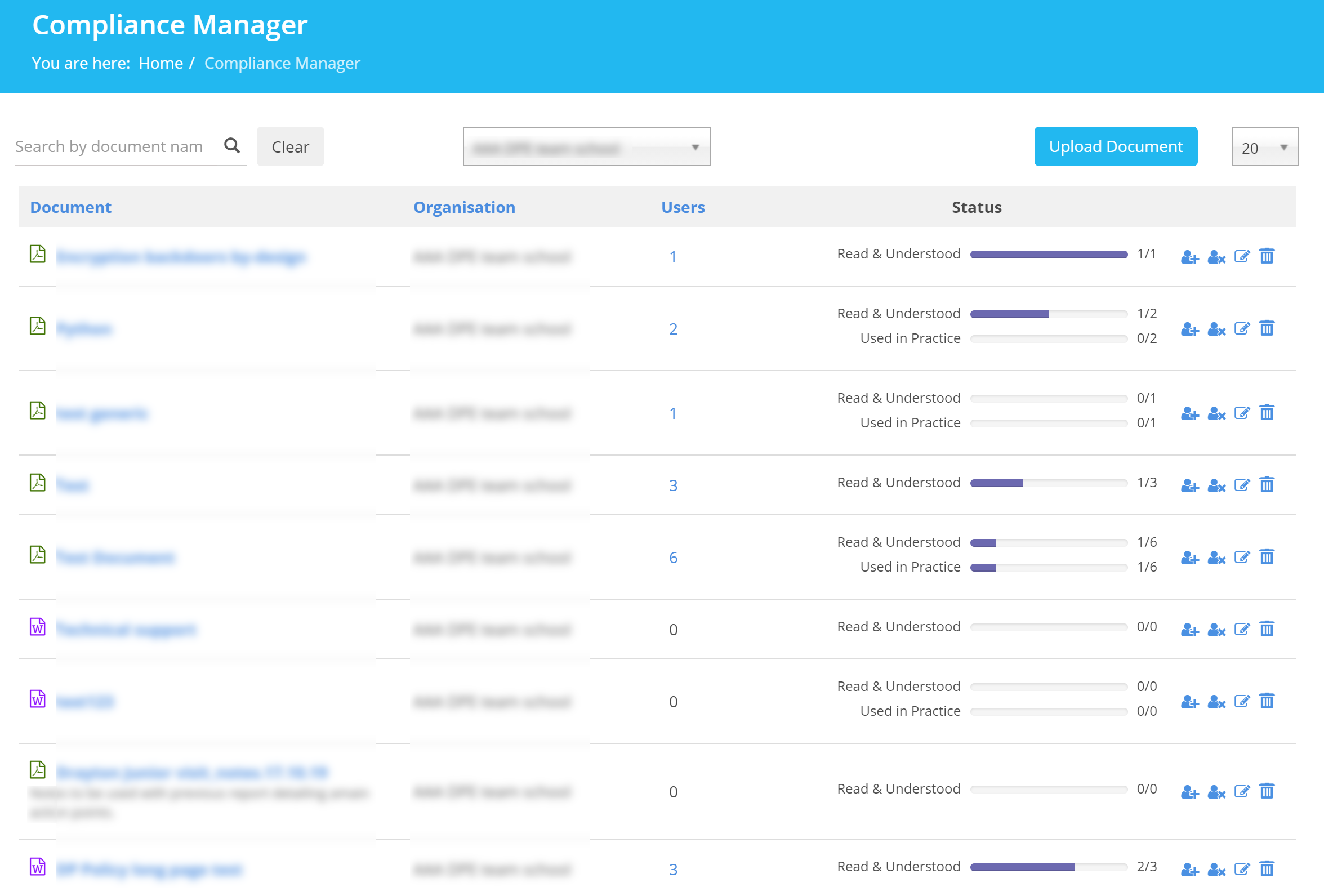Screenshot of a computer program titled “Compliance Manager” operating on a device in landscape mode. The interface features a white background with a light blue banner running across the top. The banner displays the title “Compliance Manager” in white text at the top-left corner, followed by a breadcrumb trail: "You are here: Home / Compliance Manager." Directly below this, there is a search entry field labeled "Search by document name," with a blurred-out dropdown menu next to it. Adjacent to these fields is a blue button labeled "Upload Document" and another dropdown menu displaying the number "20."

The main area of the screen is dominated by a censored list of documents, making specific details unidentifiable. Information about the organization is also blurred out. Several rows indicate the number of users (ranging from 0 to 6) and their status, including categories like "Read and Understood" and "Used in Practice," each represented by a purple bar graph. Adjacent to these graph bars are four small blue icons per line, their precise functions obscured due to the censorship. The overall color scheme combines white, light blue, gray, and a touch of purple, providing a clean and organized look to the interface.